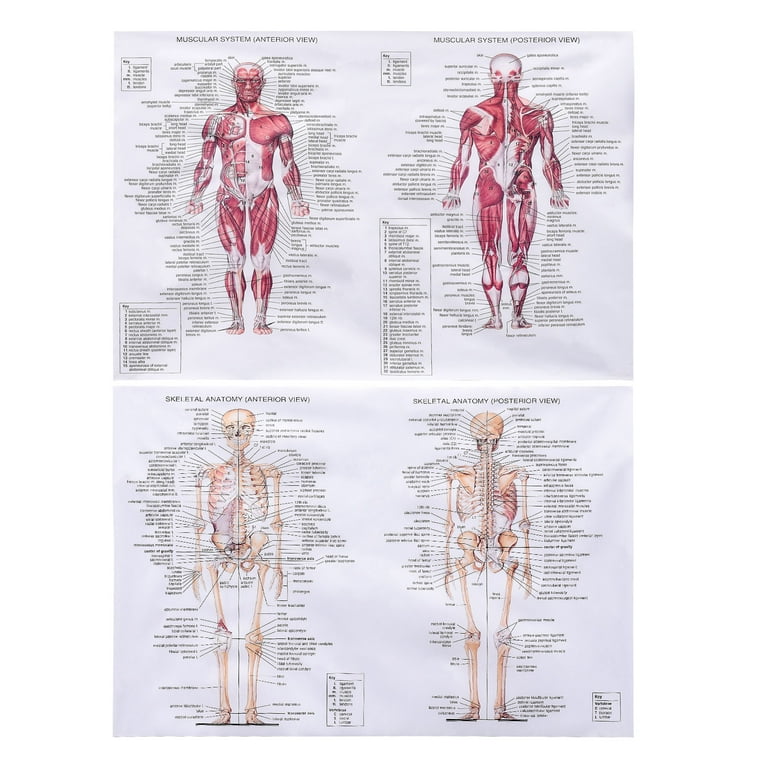The image depicts two distinct educational posters. The upper poster illustrates the muscle groups of the human anatomy in meticulous detail, both from frontal and dorsal viewpoints. It presents an x-ray-like view of a person devoid of skin, thereby revealing the intricate network of muscles. Each muscle group is carefully labeled, providing specific names and detailed annotations to facilitate anatomical study.

Beneath this, the second poster focuses on the human skeletal system, presenting a comprehensive diagram of human bones. This poster highlights the complete skeletal structure without any overlay of muscles, making it easier to identify individual bones. Similar to the muscle poster, this diagram features numerous labels for each bone, emphasizing the complexity and intricacies of the human skeletal framework. Both posters serve as valuable resources for understanding human anatomy, with clear and detailed labels that support educational and reference purposes.